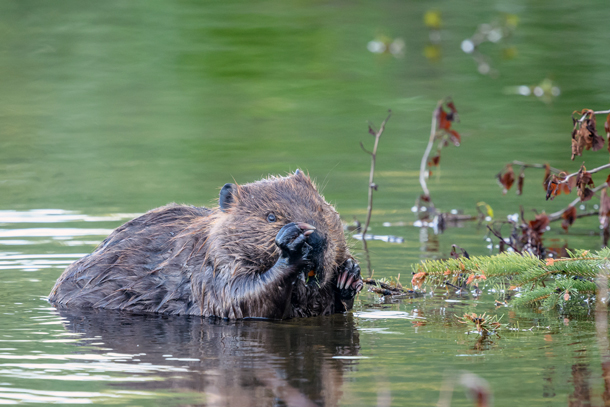The zoomed-in image captures a beaver, partially submerged in a body of greenish water, possibly a lake, pond, or marsh. On the left side, the brown beaver is depicted with its claws near its face, as if rubbing or holding something close to its mouth, showcasing its sharp nails, small brown eyes, and two front teeth. Its fur appears matted and wet. Surrounding the beaver, on the right, are sparse plant life with twigs and branches emerging from the water. These branches lack lush foliage, with some bearing brown, withered leaves, indicative of autumn or winter. At the bottom right corner, Christmas tree-like branches, possibly part of the embankment, protrude towards the water, further emphasizing the seasonal desolation. This detailed composition highlights the beaver amidst a tranquil yet lifeless aquatic environment.